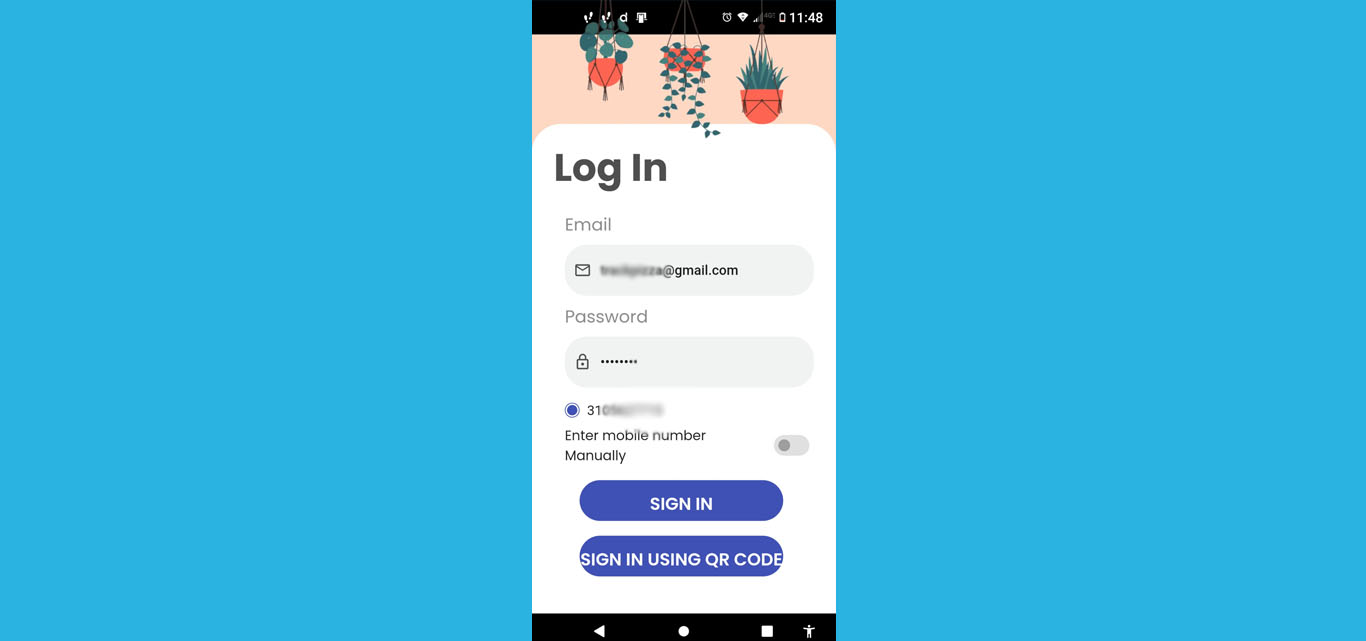The image showcases a detailed screenshot of a phone with a blue background to the left and right. The screenshot is centered and features a black status bar at the top. Within this bar, there are four indistinct icons on the left, resembling footprints, a lowercase "d", and small squares. Moving right, the bar displays icons representing an alarm clock, a diamond, cell signal bars, a battery indicator, and the time, 11:48 AM.

Overlaid in front of this status bar are three hanging potted plants. The first, on the left, is in a pink pot with three tassels and nine green money plant leaves. The second plant also occupies a pink pot and features three hanging strands with a long vine. The third plant is a green succulent, housed in a similarly styled hanging pot, with two tassels and a single attachment point, set against a tan or peach background.

Below these plants, the interface transitions to a white background with black text. It prominently displays the login area. The text reads "log in," followed by sections for "email" and "password." The email field features a gray envelope icon and has an email address partially visible, ending in "@gmail.com." The password field shows a gray lock icon with obscured password characters.

Further down, there's a selectable purple circle marked "31" with some blurred content, and a prompt in black text to "enter mobile number manually," which hasn’t been selected and is grayed out. The interface then shows two buttons: one purple button with white text reading "sign in" and another reading "sign in using QR code."

Finally, at the bottom of the screen, a black bar contains icons in white: a play button (triangle), a circle, a square, and a silhouette of an individual.